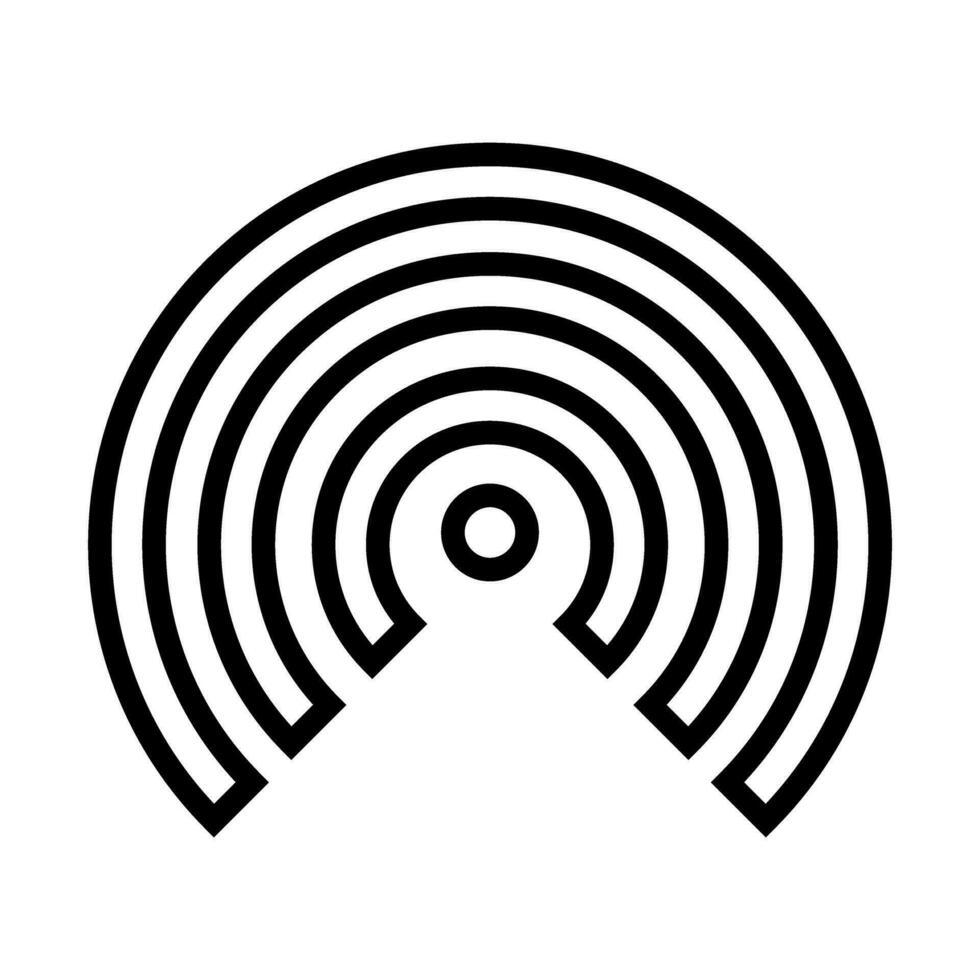The image resembles a captivating optical illusion or maze, characterized by a series of three concentric arcs that create a mesmerizing visual effect. Each arc forms three-quarters of a circle, squared off at the bottom and outlined in a thick black line, with a stark white interior. These arcs encircle a small, central round circle, which features a dot in its center. The bottom of the image, making these arcs appear as if they are floating above a continuous road, leads to the middle circle. This structured arrangement of arcs and circles, with its heavy black outlines, evokes a sense of wonder and can be interpreted as various forms, ranging from an incomplete keyhole to an amphitheater. The optical illusion lies in the way the lines flow seamlessly from the outer arcs to the center, creating a complex and thought-provoking visual experience.